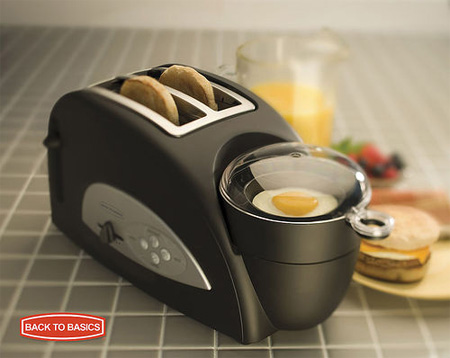The image depicts a compact, multi-functional black toaster with a distinctive half-arch rounded top. The left side of the appliance features a chrome-colored section equipped with a black knob and four adjacent silver buttons. Two halves of an English muffin are toasting at the top, while a glass-covered egg poacher at the front is cooking an egg, its yolk clearly visible. The toaster sits on a gray tiled surface adorned with tiny, uniformly spaced tiles accented by white lines. To the right of the toaster, there’s a pitcher partially filled with orange juice and a plate with an assembled English muffin sandwich, containing meat, cheese, and egg. Out of focus in the background, a bowl of strawberries and blueberries is visible. In the bottom left corner, a red oval emblem with a white outline and text reads "Back to Basics."